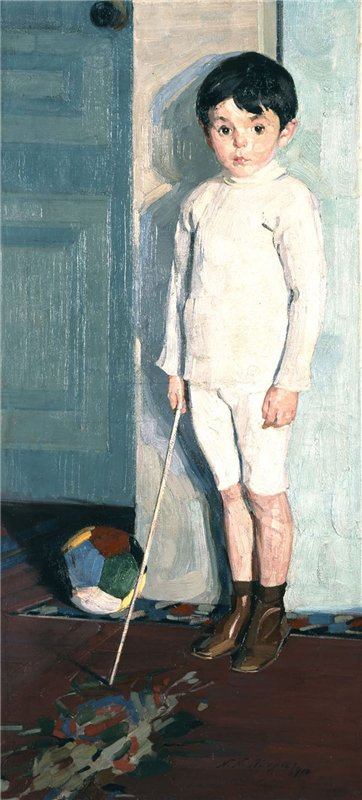The painting depicts a young boy, approximately seven or eight years old, standing in front of a white wall. He has short black hair and black eyes, and his fair skin contrasts with his dark features. The boy is wearing a white long-sleeved shirt, white shorts or bloomers, brown socks pulled up past his ankles, and brown shoes. He is holding a thin white stick in his right hand, which is pointed towards the floor. On the floor near him, an abstract collection of splotches in reds, blues, greens, and grays suggests a spill of some kind. Behind him, slightly to the left, there is a multi-colored, multi-paneled soccer ball featuring yellow, blue, red, green, white, and black sections. He stands in front of a white door with a doorknob, which is just above his eye level. The floor beneath him is a maroon color with a signature, too faded to read, written in black. The whole scene appears to take place indoors, possibly in a hallway or room.